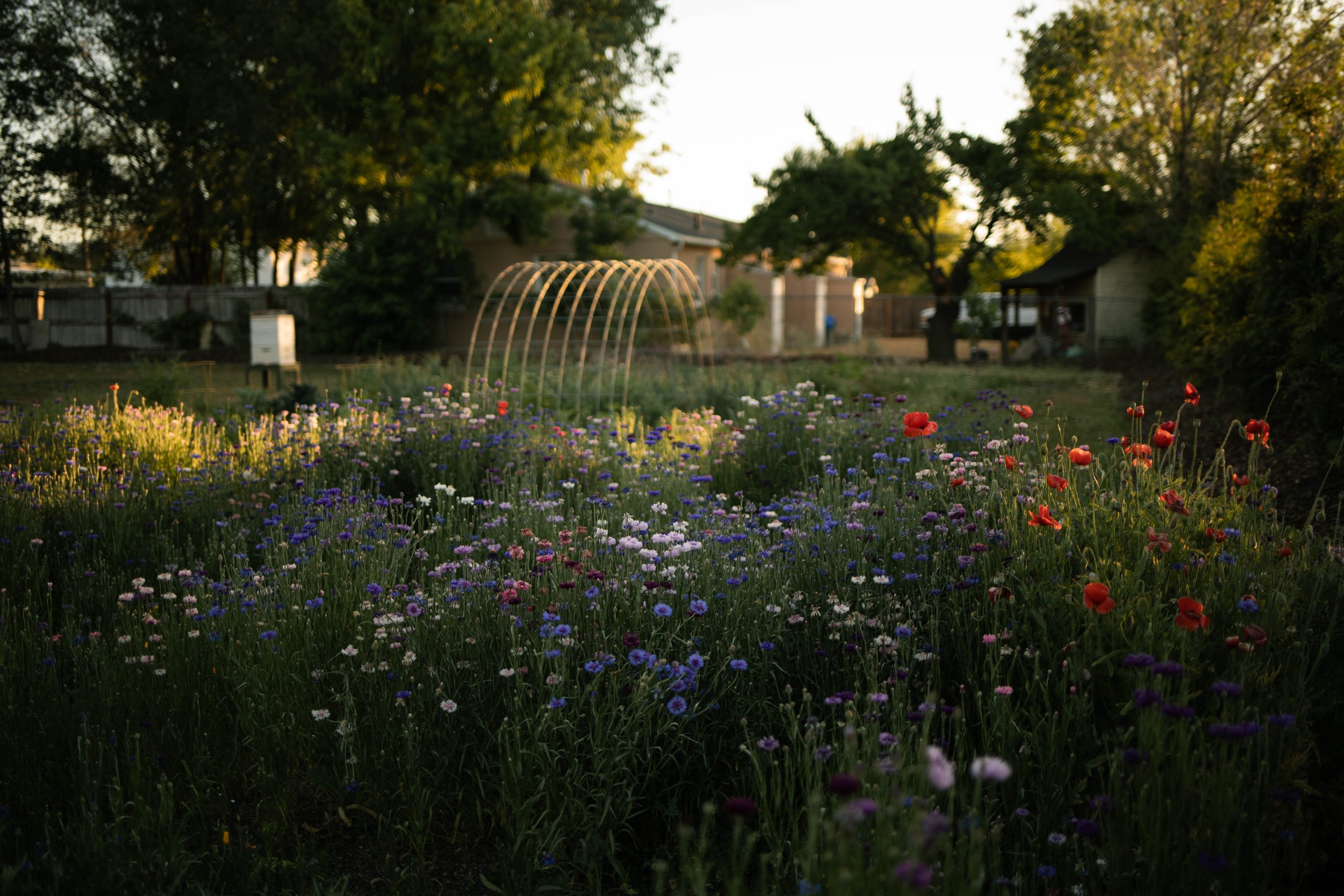A vibrant color photograph captures a lush field of tall wildflowers in the foreground, showcasing a stunning array of colors, including red, blue, white, yellow, orange, purple, pale lavender, pink, and maroon. The flowers, identified as varieties such as California poppies and bachelor buttons, grow in clusters that create a rich tapestry of hues against green stems. In the middle ground, a metal semicircle, resembling a trellis or garden hoop, stands without any coverings, hinting at its potential use for supporting vines in a tunnel-like structure. To the left, about 100 to 200 feet in the background, there is a tall, square-shaped box, possibly a bee box, elevated on a four-legged table. The surrounding yard features grass, and further back, there is a wooden fence stretching across the scene. On the right side, and enveloping the entirety of the upper part of the image, several trees frame the setting, with a particularly large tree and a building, likely a home, visible behind the fence. The photograph appears to be taken during twilight, either at sunrise or sunset, under a clear sky, adding a serene and calming tone to the landscape.